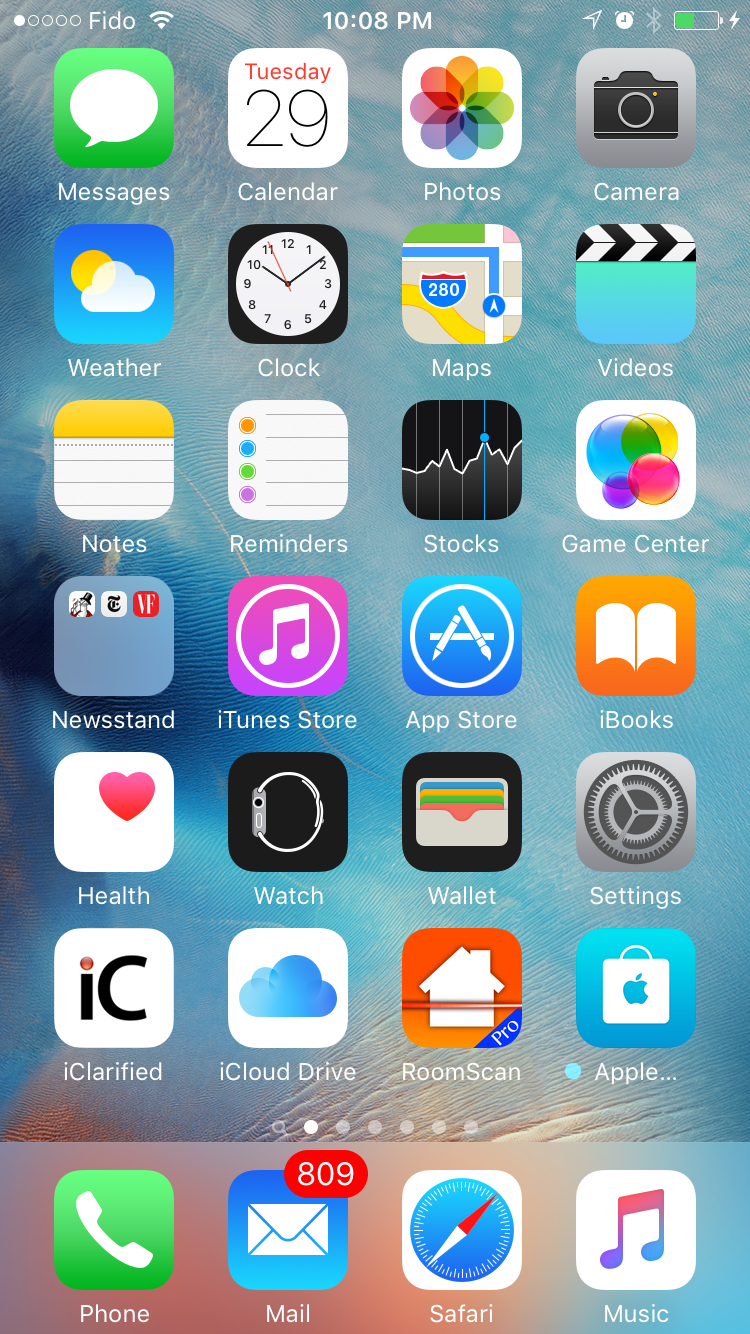The image depicts a smartphone screen displaying various details and app icons. The top left corner indicates the carrier as "Fido," and the time shown is 10:08 PM. The battery icon suggests approximately 50% charge remaining. The screen features six rows of app icons, arranged in a grid of four per row, each labeled with the respective app's name. The apps, listed from top left to bottom right, are: Messages, Calendar, Photos, Camera, Weather, Clock, Maps, Videos, Notes, Reminders, Stocks, Game Center, Newsstand, iTunes Store, App Store, Books, Health, Watch, Wallet, Settings, Clarified, iCloud Drive, Room Scan, and Apple. At the very bottom, four additional app icons are positioned: Phone, Mail, Safari, and Music. Notably, the Mail app icon has a red notification badge in the top right corner, indicating 809 unread messages.